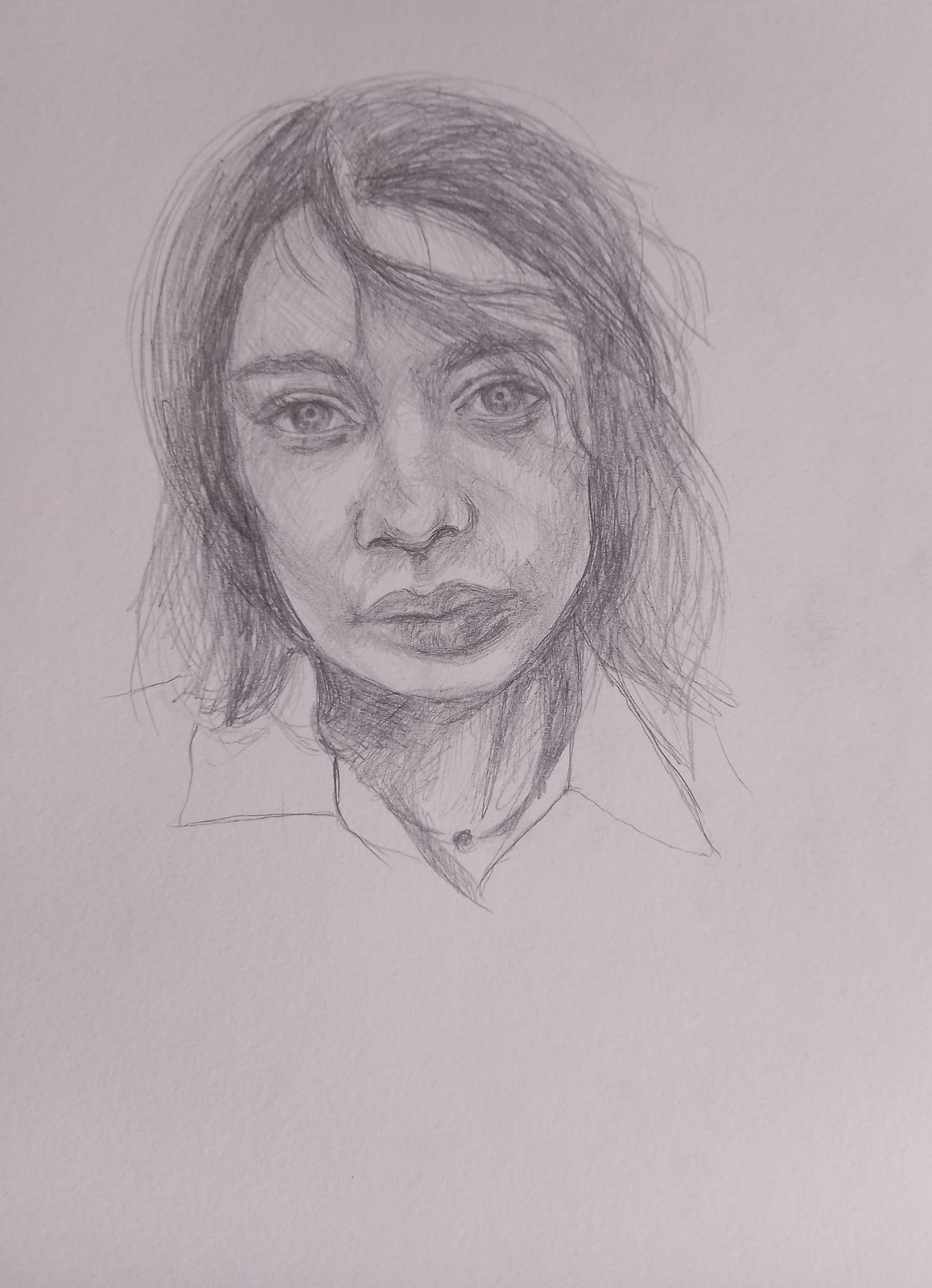This detailed caption provides a comprehensive description by integrating the shared details from all three voices:

The image is a photograph of a pencil sketch drawn on a white piece of paper, appearing gray due to the lighting. It portrays a young woman, possibly in her late 20s or early 30s, with an ambiguous racial appearance. She has slightly African-American features but straight hair that is lightly unkempt, with a strand falling across her forehead. Her oval-shaped face exhibits a serious expression with bleak, empty eyes, defined by almond-shaped pupils, prominent eyelashes, and bold eyebrows. 

Her full nose and thick lips, which nearly reach her chin, are depicted with careful shading, showcasing the artist's skill. Her straight hair, parted on the side, reaches about shoulder length and exhibits a slight flyaway look. She wears a blouse with a sharp triangular collar and a neckerchief or bandana that comes to a point. The sketch lacks any background or text, putting full emphasis on the woman's intricately detailed face and neck.